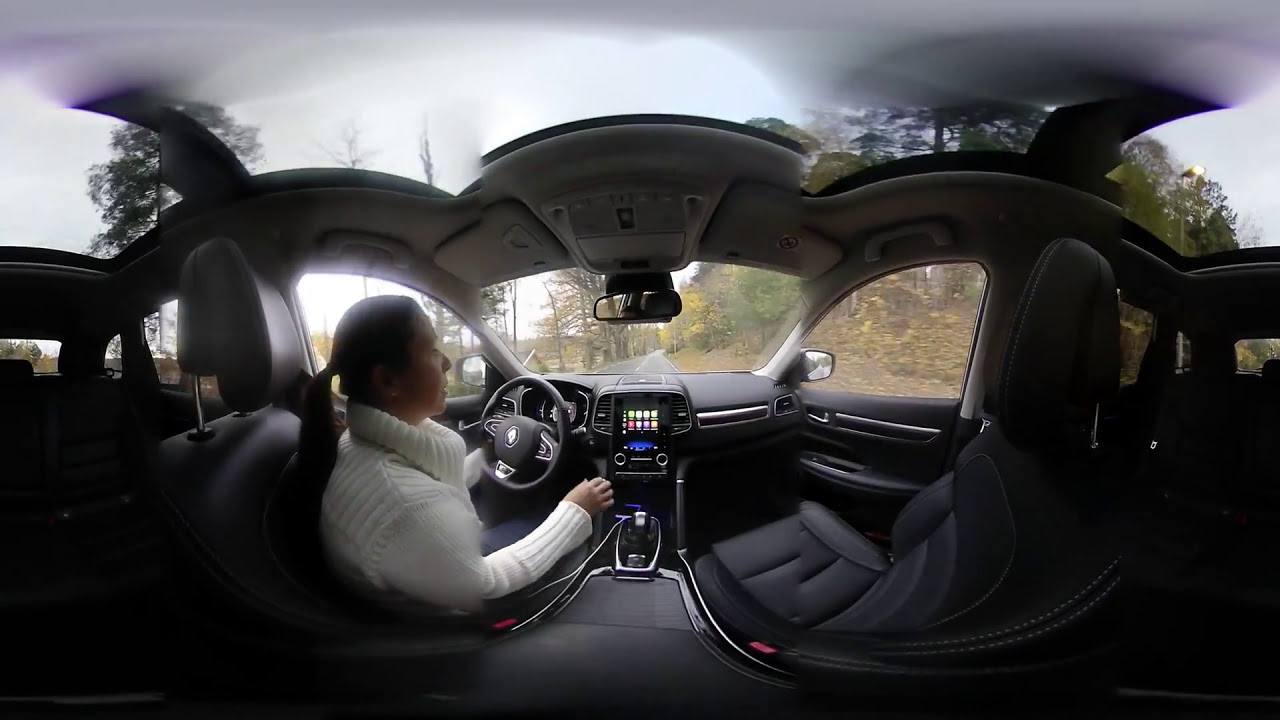The image, captured with a fish-eye lens from the backseat of a car, showcases a modern, luxury vehicle, likely a European brand, with a black leather interior. The spacious vehicle, possibly an SUV, features a sleek dashboard with a touchscreen console, fabric seating, and a black steering wheel. A woman, appearing young and petite, is driving. She is dressed in a white, long-sleeved turtleneck sweater and has her long, dark hair pulled back in a ponytail. She is focused on the road, which curves to the right in the distance. The road is lined with trees whose leaves have turned yellow, indicating fall, and the overcast sky adds to the autumn feel. The car's sunroof or moonroof allows a view of the gray sky and the tops of the trees, illuminating the otherwise empty vehicle.